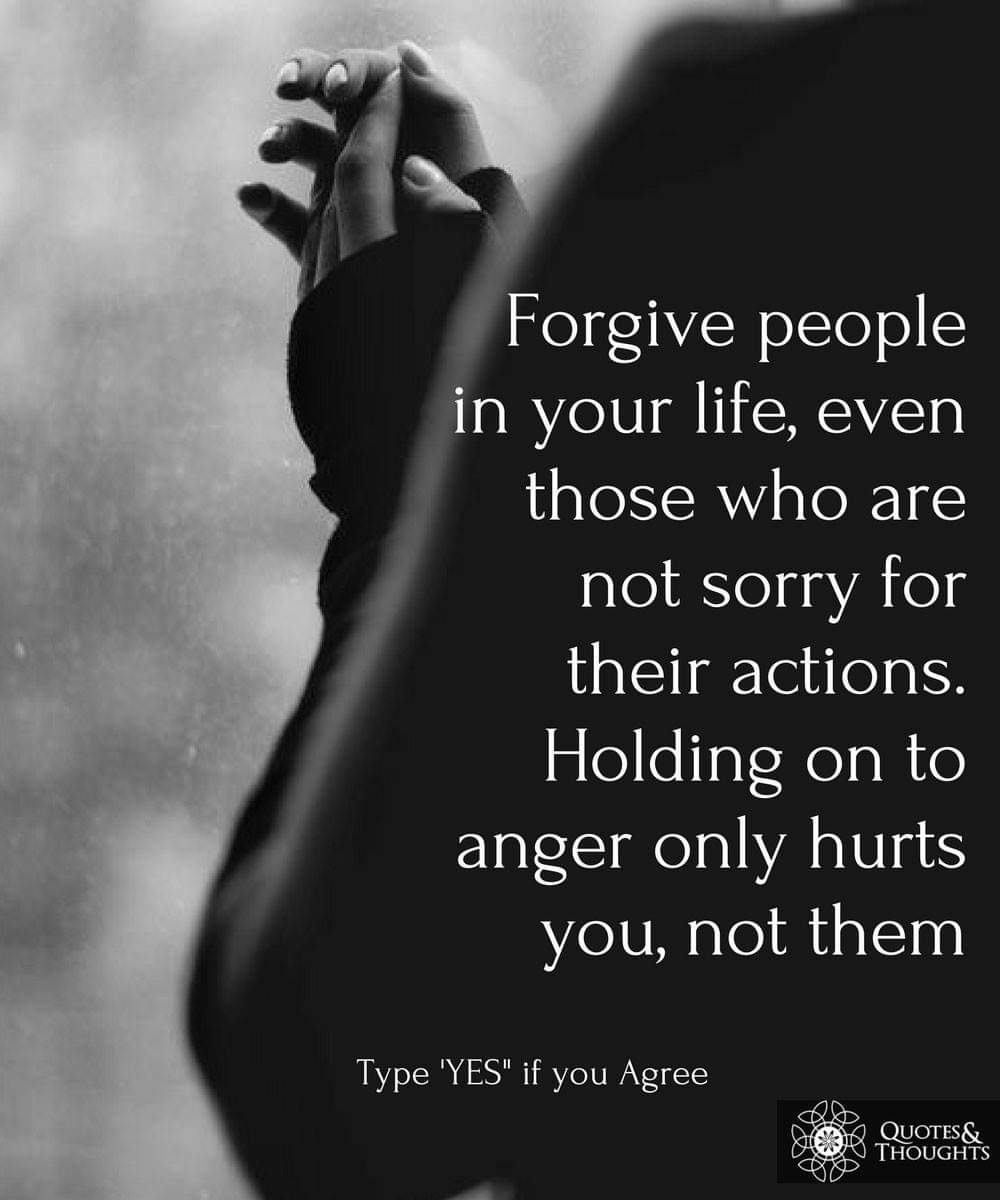This is a black-and-white poster featuring a thoughtful quote overlaying a blurred image. The main subject appears to be a woman, viewed from behind her left shoulder, dressed in a long-sleeved shirt that covers her knuckles. Her hands are positioned together as if in prayer, creating a contemplative mood. The background is a fuzzy black and gray, enhancing the somber and introspective tone of the poster. The quote, rendered in white text, reads: "Forgive people in your life, even those who are not sorry for their actions. Holding onto anger hurts you, not them." Below the main quote, it prompts the viewer with, "Type yes if you agree." In the bottom right-hand corner, the icon and text "Quotes and Thoughts" are displayed, adding a finishing touch to the composition.